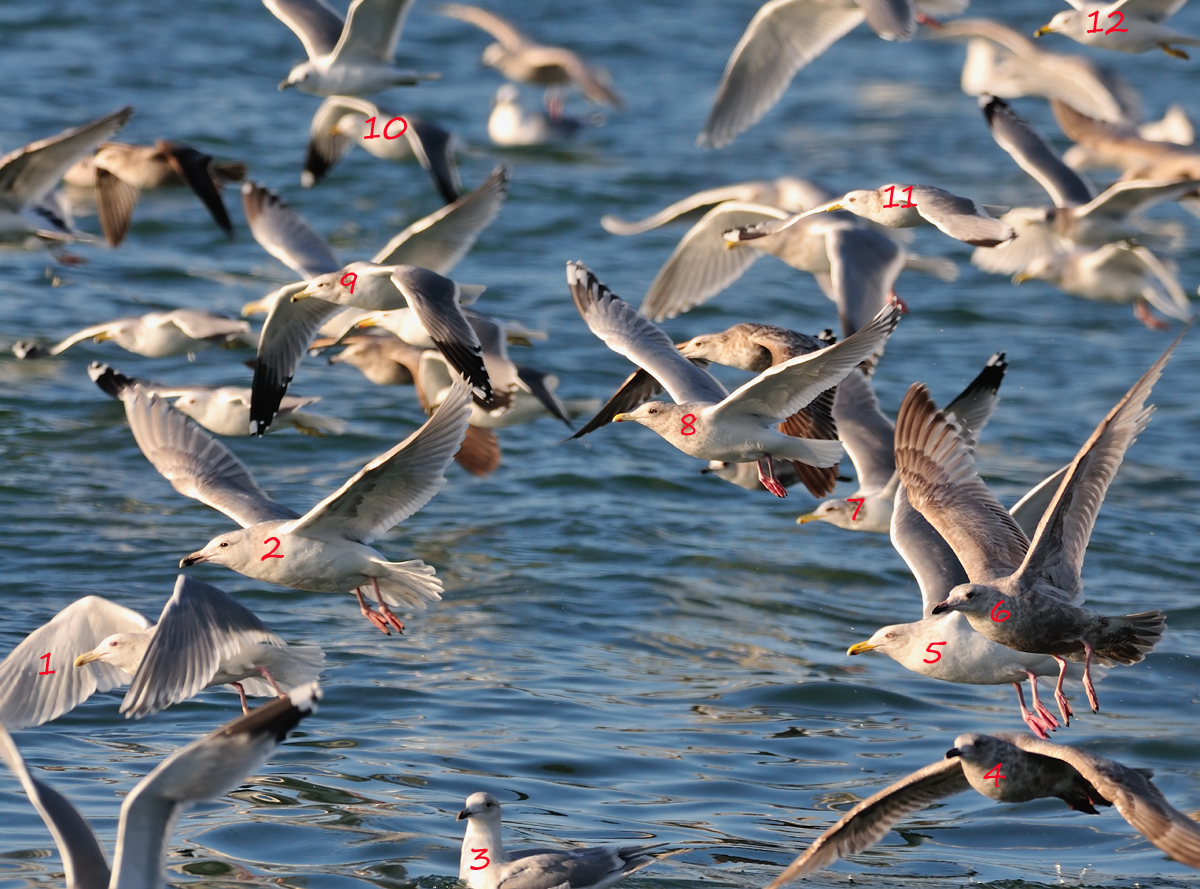A digital photograph captures a dynamic scene of seagulls over an expansive body of blue water, which is slightly choppy. The image features a mix of approximately 20 seagulls, differentiated by varying degrees of clarity and motion. In the foreground, 12 seagulls are visibly numbered in red ink, distributed as follows: Seagull 1 is near the bottom left corner, Seagull 2 just below Seagull 9, Seagull 3 is left of the center at the bottom in the water, Seagull 4 is almost at the bottom corner, Seagulls 5 and 6 are at the bottom right, Seagull 7 is just to the bottom right of Seagull 8, Seagull 8 is to the bottom left of Seagull 11, Seagull 9 is directly under Seagull 10, Seagull 10 is more towards the central-left, Seagull 11 is situated in the right center, and Seagull 12 is in the upper right of the frame. The seagulls exhibit diverse behaviors; some are in flight, wings flapping, while others are bobbing on the water or sitting with wings tucked. The majority of the unnumbered seagulls, which add to the flock's total, are scattered throughout the scene, further emphasizing the bustling activity. The composition is striking, with a notable gap in the middle of the frame devoid of any birds, and a still lake that gives a serene backdrop to the lively avian spectacle, hinting at the time of sundown with a subtle atmospheric glow.